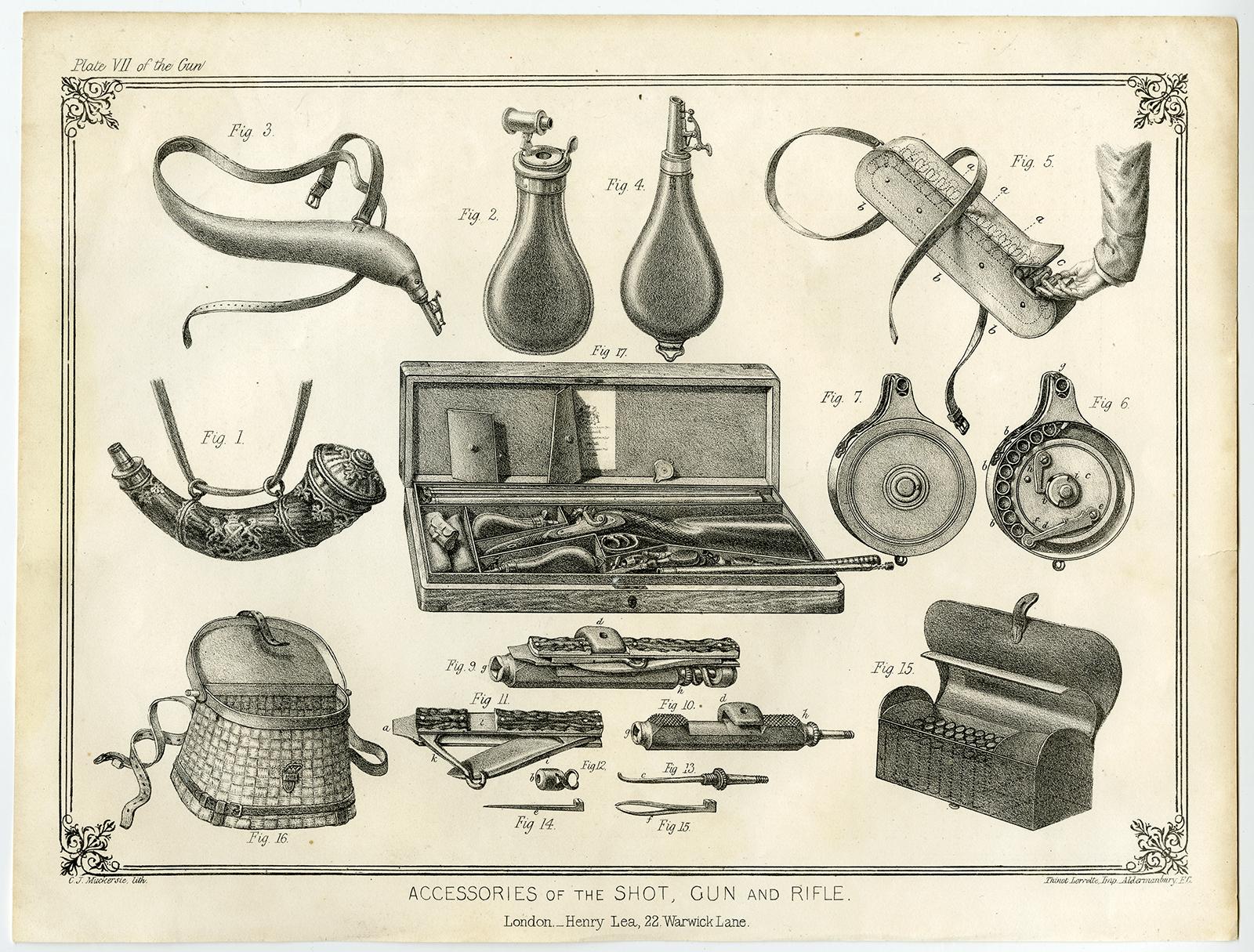This detailed illustration, likely from the 1800s, is titled "Accessories of the Shot, Gun, and Rifle" and is credited to London Henry Lee, 22 Warwick Lane. The aged paper has a yellowish tint and features intricate, pencil-drawn images enclosed in a black-bordered frame. In the center, a wooden case is displayed; it contains a disassembled rifle with its butt and barrel neatly placed in compartments, along with various other accessories. Surrounding this case are multiple labeled figures showcasing additional accessories. Figure 1 appears to be an intricately designed gunpowder horn, possibly made from an ivory tusk with metal fittings. Above it is a leather-like tube, likely another gunpowder container. Other figures include leather bulbs, possibly for holding shot or ammunition, a belt with compartments for individual shells, and an ammunition canister reminiscent of those used for automatic firearms. The highly detailed drawings and period-piece elements suggest the image is indeed quite old, giving us a glimpse into the firearm accessories of that era.